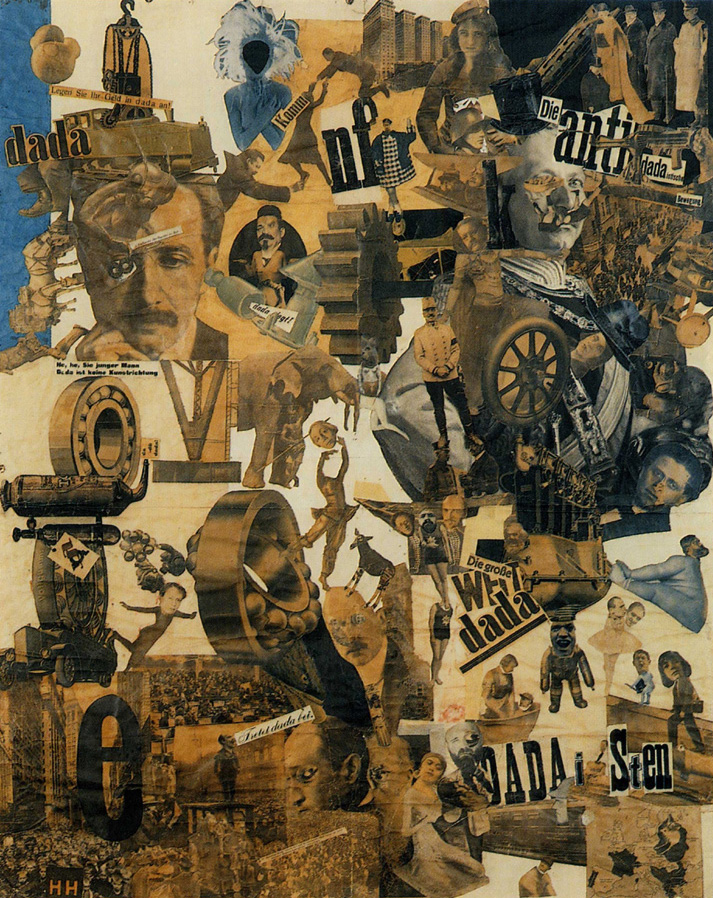This image is a complex and detailed collage predominantly featuring a yellowish-brown aesthetic, with subtle hints of blue scattered throughout. Composed of numerous magazine clippings, the collage primarily showcases images of men from older times, evoking a sense of historical depth. At the top left, the word "Dada" is prominently displayed, setting a possible thematic tone related to the Dada art movement. Further inspecting the collage reveals labels with letters such as "Di Anti Dada," "F," an "E" in the bottom left corner, and "HHs".

The middle section features a dynamic and surreal vignette of a woman and a man suspended in the air, reinforcing the eclectic and avant-garde nature of the composition. The bottom left corner depicts an urban landscape teeming with buildings and a bustling crowd, adding a sense of scale and context. Furthermore, scattered throughout the image are various references to military and political themes, including old photographs of men in military gear and glimpses of ammunition, suggesting a historical or socio-political commentary embedded within the collage.